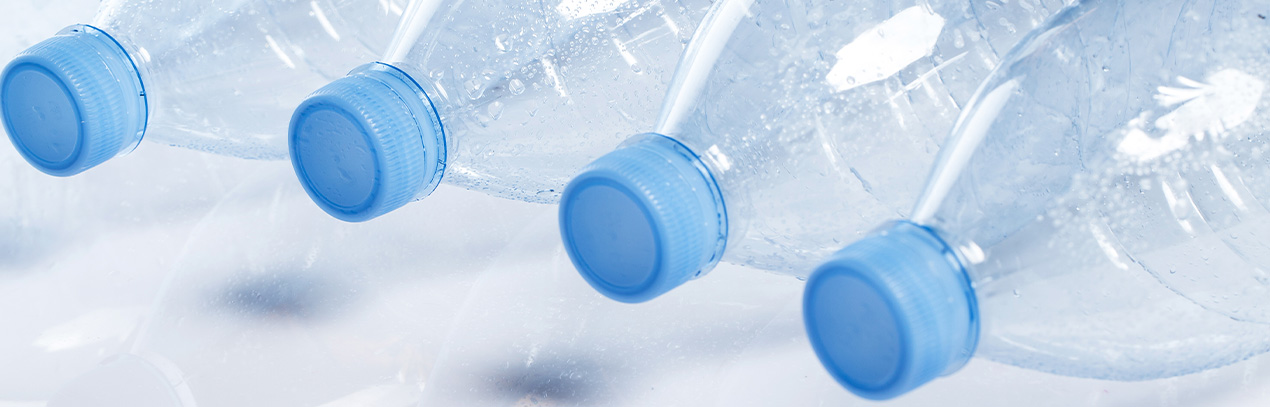This is a close-up, horizontally rectangular photograph capturing four identical plastic bottles arranged in a row, seen predominantly from the top portion. Each bottle features a blue twist-off cap that is securely closed, and they are all clear and devoid of labels. The transparent bodies of the bottles showcase visible water droplets, suggesting they have been in contact with moisture. The image, taken indoors, includes a greyish background with darker spots, though the primary focus remains on the bottles. The surface they are positioned on appears wet, further emphasizing the presence of water. Additionally, the lighting in the room casts a noticeable glare and shadows on the necks and lids of the bottles, enhancing their three-dimensional appearance. The bottles are sleek, featuring the typical vertical ridges common to many plastic water bottles.